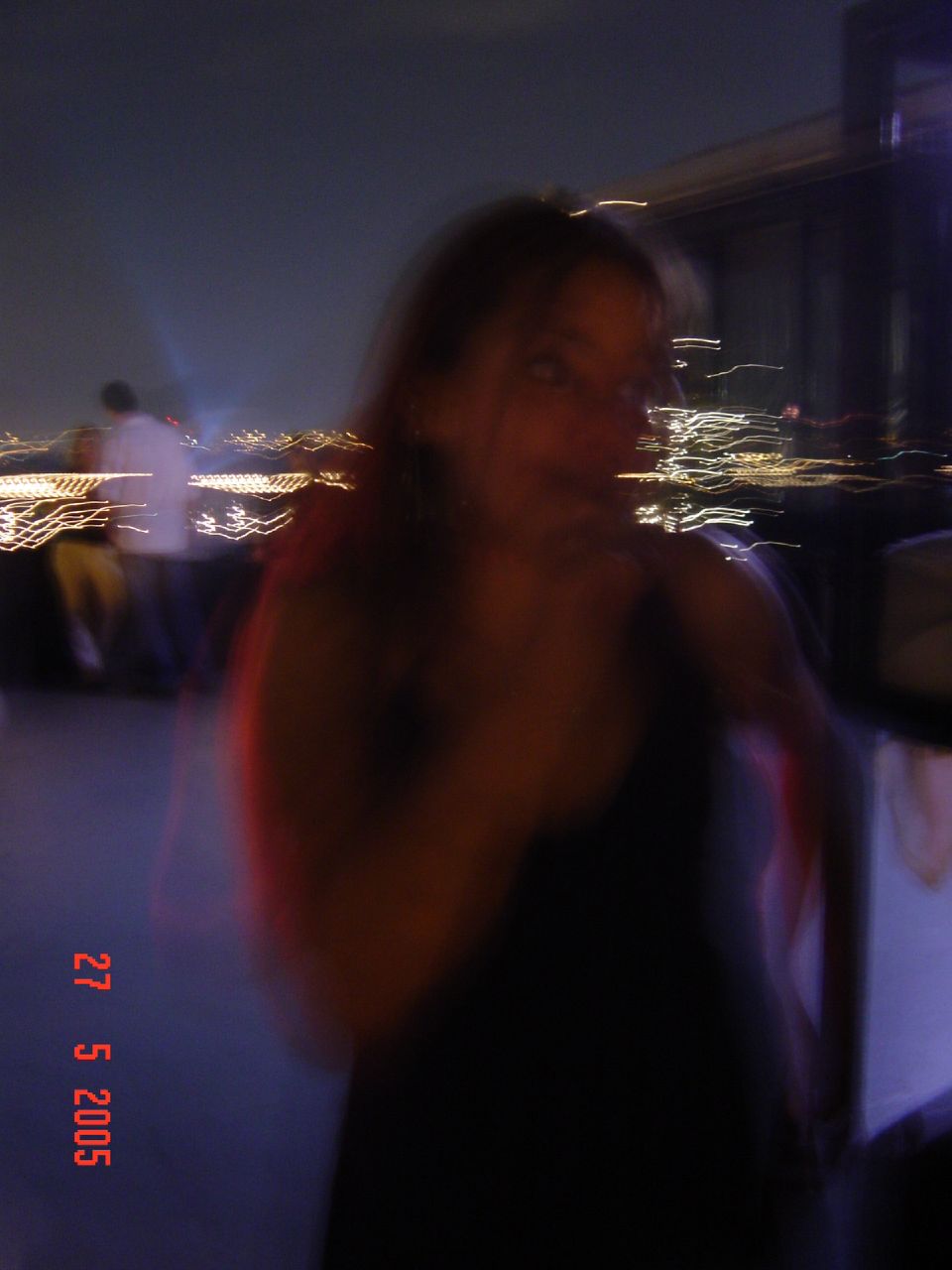The photograph, taken at night and heavily blurred, captures an outdoor scene that appears to be on a balcony or rooftop with a city skyline in the background. The dark sky fades into a slight blue, punctuated by squiggly lines of city lights on the horizon. In the forefront stands a woman in a dark, possibly sleeveless dress, her long dark hair swept to the side. She is leaning against a doorway or doorframe, with her left hand behind her and her right hand raised to her mouth, as if holding or doing something, though it’s not discernible due to the blur. Over her left shoulder on the left side, there are two figures, a man and a woman, standing close together and seemingly gazing out over the edge. A red date stamp in the bottom left corner reads "27-5-2005."